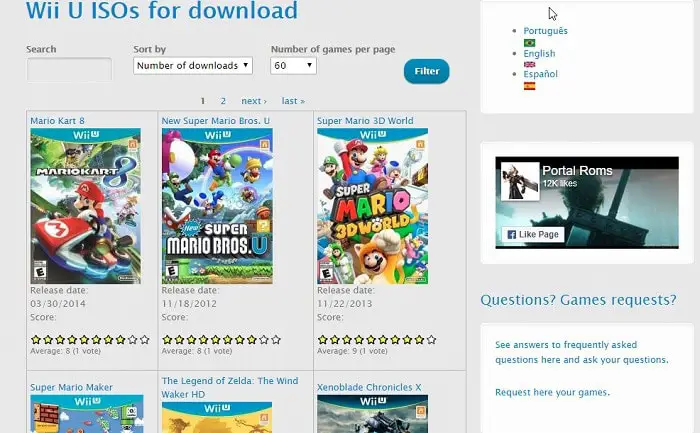This image portrays the homepage of a web store dedicated to game downloads. At the very top of the page, a prominent blue banner reads, "We use ISOs for download." Directly below, on the left side, there is an empty search bar for users to find specific games. Next to it is a dropdown menu labeled "Sort by," with an option to sort by "number of downloads." To the right of that is a customizable feature for displaying the "number of games per page," currently set at 60, followed by a blue "Filter" button.

On the far right, there is a language selection section featuring three flags: the Brazilian flag for Portuguese, the UK flag for English, and the Spanish flag for Español. Below this is a tab labeled "Portal," adjacent to a promotional video trailer for "Final Fantasy 7."

Further down, the sections labeled "Questions," "Games," and "Requests" are visible, with links to "see answers to frequently asked questions here" and to "ask your questions" or "request your games."

The main content area is presented like a storefront, showcasing several game titles. Featured prominently is "Mario Kart 8" with its cover art, a release date of March 30, 2014, and a rating of 8 stars. Other visible titles include "Super Mario Bros Wii," "Super Mario Bros U" for Wii U (release date November 18, 2012, 8 stars), and "Super Mario 3D World" (release date November 22, 2013, 9 stars).

The top edges of additional game covers are barely visible at the bottom of the image, hinting at titles such as "Super Mario Maker," "The Legend of Zelda: The Wind Waker," and "Xenoblade Chronicles X." However, only the upper portions of these covers are in view, suggesting the image might have been cropped.